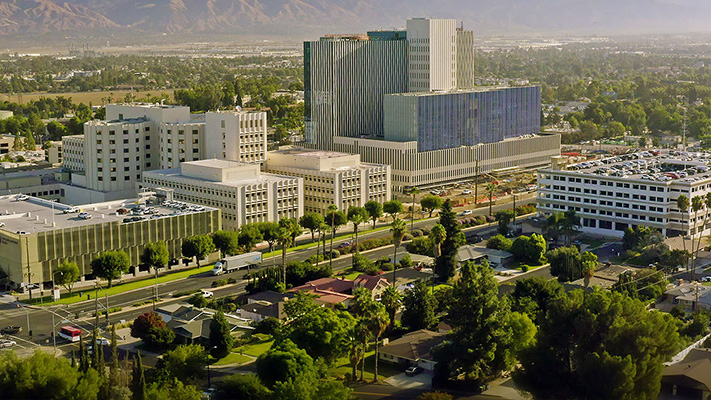This is an aerial photograph capturing a bustling cityscape characterized by a mix of buildings. Dominating the image are square and rectangular office buildings and possibly a factory, all distinctly white and composed of concrete. There’s a prominent parking garage on the right, with 30-50 cars visibly parked on its roof. A key highlight is the vibrant greenery, with trees scattered extensively throughout the scene, lining the streets and dividing the wide, four-lane road that runs through the area.

In the foreground, smaller structures and homes are nestled among the trees, surrounded by sectioned-off areas. Old cars can be seen along the meandering streets, adding to the lively city atmosphere. The streets are notably lined with trees, enhancing the overall verdant aesthetic.

The photo, taken in possibly spring or summer, shows everything from a horizontal perspective. At the top of the image, a hazy horizon unveils flat lands, eventually transitioning into brown, mountainous structures reminiscent of the landscapes around Phoenix. This detailed capture highlights the contrast between the rigid urban setup and the lush, surrounding greenery.